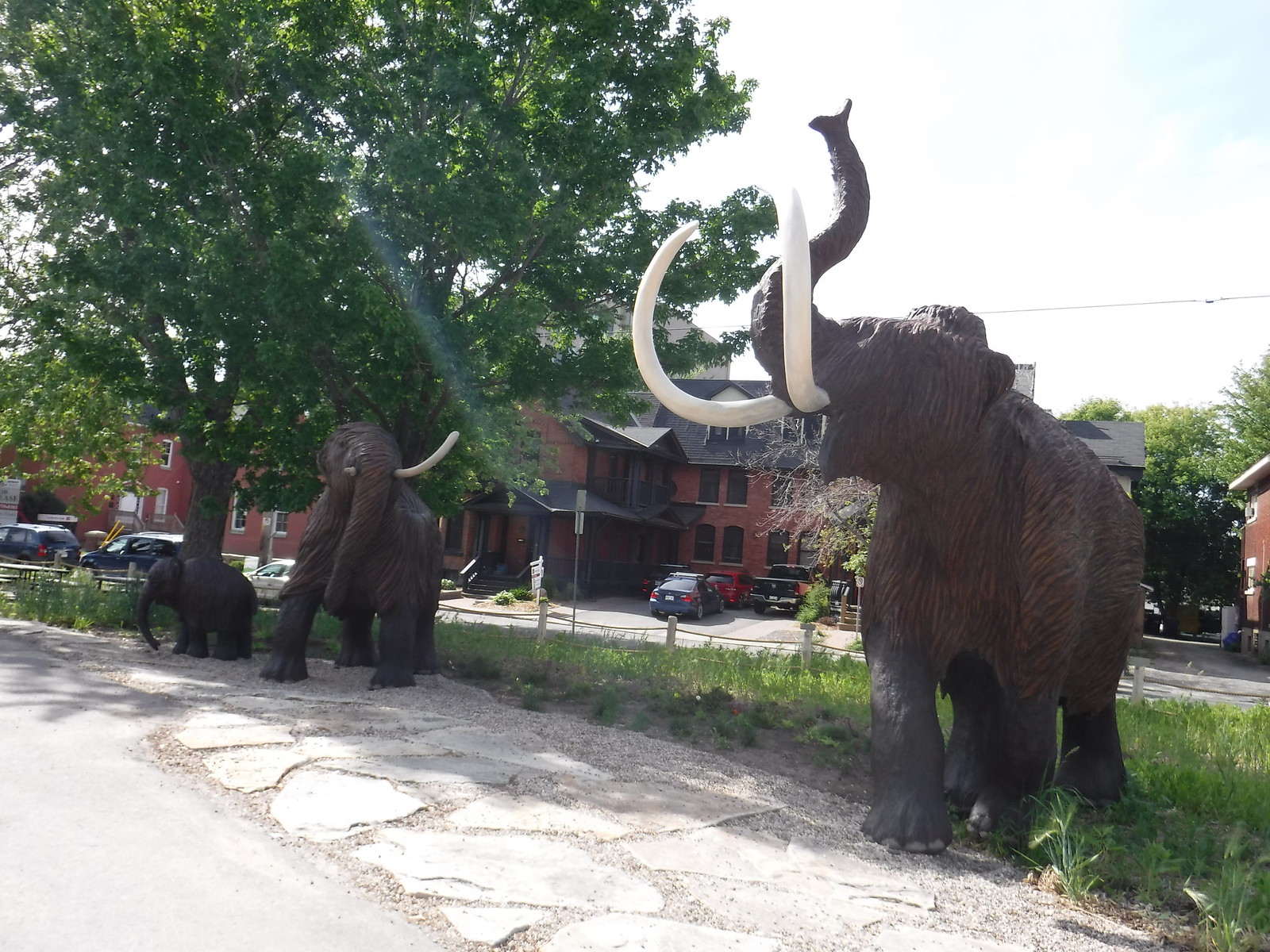The photograph captures an outdoor daytime scene in bright light, possibly in a foreign country, featuring three sculptures of woolly mammoth elephants. The largest mammoth is positioned closest to the right side, standing partly on a white stone walkway and partly on a grassy area, with its head and trunk raised, and two curled white tusks prominently visible. To the left, slightly in the background, a medium-sized mammoth, possibly the female, also displaying two tusks, though one appears to be missing. Between them stands a smaller mammoth, likely a baby, under a large, leafy tree. The scene is framed by a chain and pole fence, beyond which a paved road runs. On the other side of the road is a red brick building with a three-story structure and two cars parked in its driveway. The foreground features a cobblestone or cut-brick path where the mammoths are displayed. The image, devoid of any text or print, is richly detailed with natural elements like grass and brick, under the direct overhead sunlight.